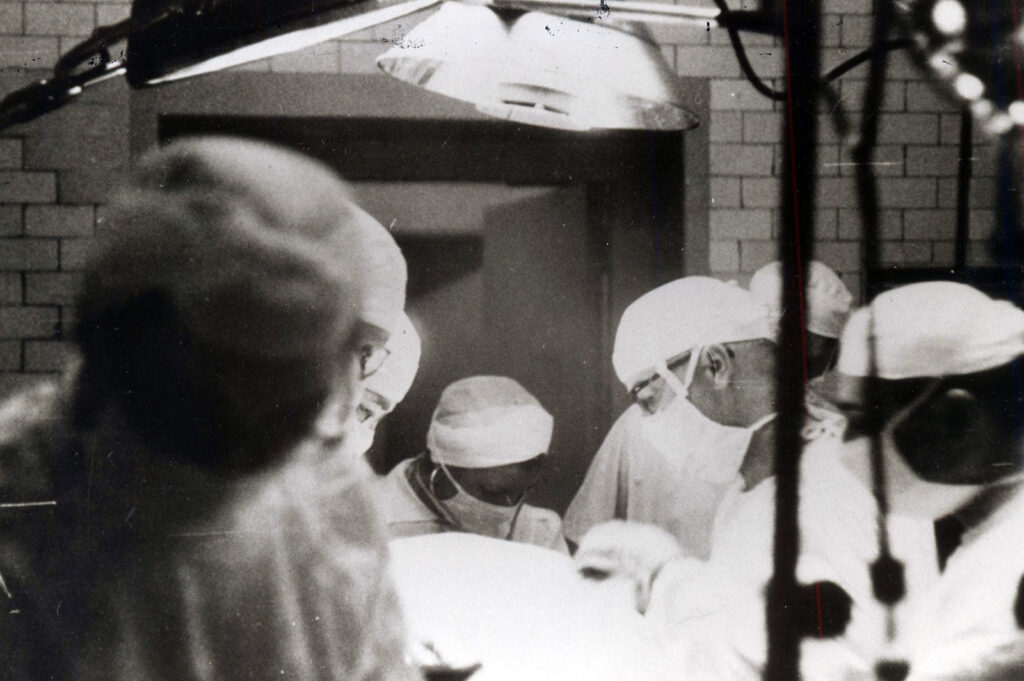The black-and-white rectangular photograph captures a vintage scene inside a hospital operation room. On the left side of the image, we see a person wearing glasses, while on the right side, a man also with glasses appears to be operating, with hands raised. The operation table is partially visible, with a patient covered by a white cloth, and a faint outline of the patient can be seen beneath. Surrounding the table are several medical professionals, dressed in white surgical outfits including masks, hairnet covers, gowns, and gloves, with one individual notably wearing a stethoscope. The backdrop features a white brick wall with marks, and an open doorway prominently positioned in the center. Overhead, several spotlights illuminate the scene, emphasizing the central white mass of the operation table. In the right area of the image, there are black stands that might be light stands. The overall ambiance suggests an intense and focused surgical procedure.